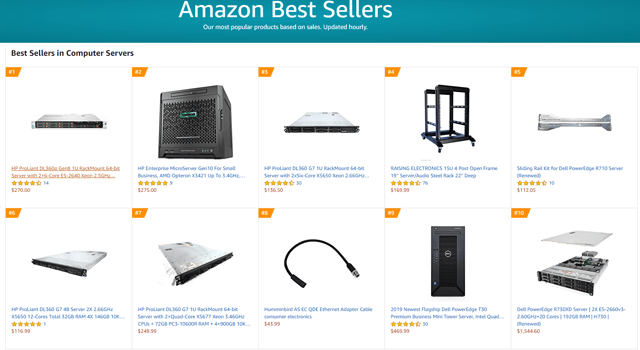The image is a screenshot of an Amazon webpage featuring a listing of computer-related products under the category "Best Sellers in Computer Servers." The top portion of the screen displays a gray gradient banner that reads "Amazon Best Sellers: Our most popular products based on sales. Updated hourly." Below this, there are visible two rows of product listings, each row containing five items, making a total of ten products.

Each product box is marked with an orange banner in the top left corner, displaying the ranking number in white text. The items range from server towers, server racks, and hard drives, to various cords such as power cords and USB cords. Notably, a power or USB cord is centered in the bottom row. The small size of the screencap makes it difficult to read the detailed text associated with each product.

Underneath each product image, links to the product pages are included, along with the star rating for reviews and the price. The layout is designed to allow easy navigation for viewers to access more detailed information and make purchases.